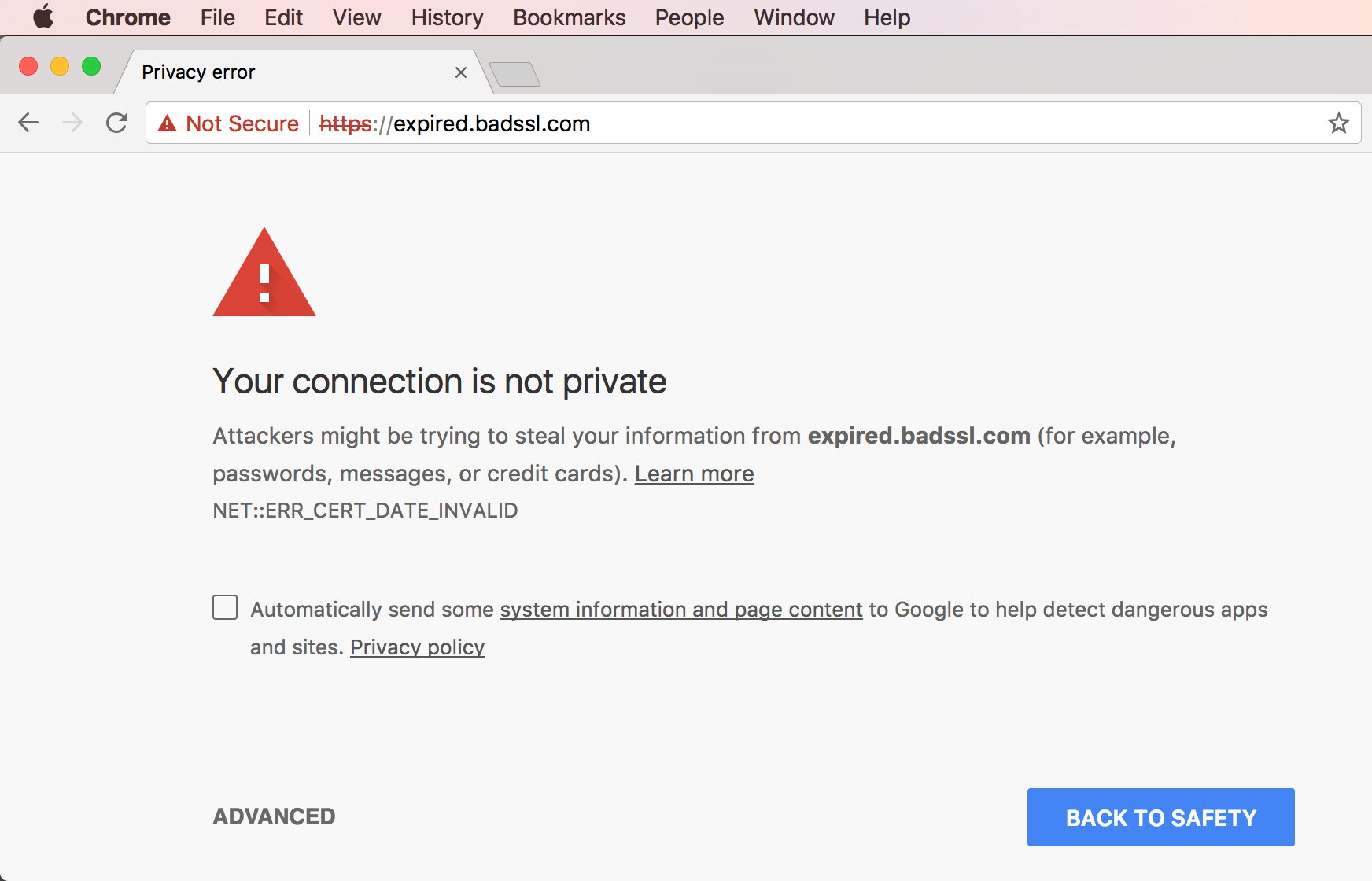The screenshot captures a Chrome browser window displayed on an Apple computer. At the top of the image is the macOS toolbar, featuring the iconic Apple logo on the far left, followed by menu options such as Chrome, File, Edit, View, History, Bookmarks, People, Window, and Help.

Below the toolbar is the browser's own interface, showcasing the three colored buttons on the upper-left corner: red for closing the window, yellow for minimizing, and green for maximizing. The browser has a single open tab labeled "Privacy Error," and the URL in the address bar is "expired.badssl.com," accompanied by a "Not Secure" warning illustrated by a red triangle with an exclamation mark.

The main content of the browser window displays a security warning page. At the top, a prominent red triangle with an exclamation mark alerts the user with the message: "Your connection is not private. Attackers might be trying to steal your information from expired.badssl.com (for example, passwords, messages, or credit cards)." 

A link labeled "Learn more" is available for additional information. An error code, "NET::ERR_CERT_DATE_INVALID," is present below this message. Additionally, there is an unchecked checkbox option that reads, "Automatically send some system information and page content to Google to help detect dangerous apps and sites."

Finally, at the bottom of the page are two buttons: "Advanced" on the left and a prominent blue button labeled "Back to Safety" on the right, providing navigation options for the user.